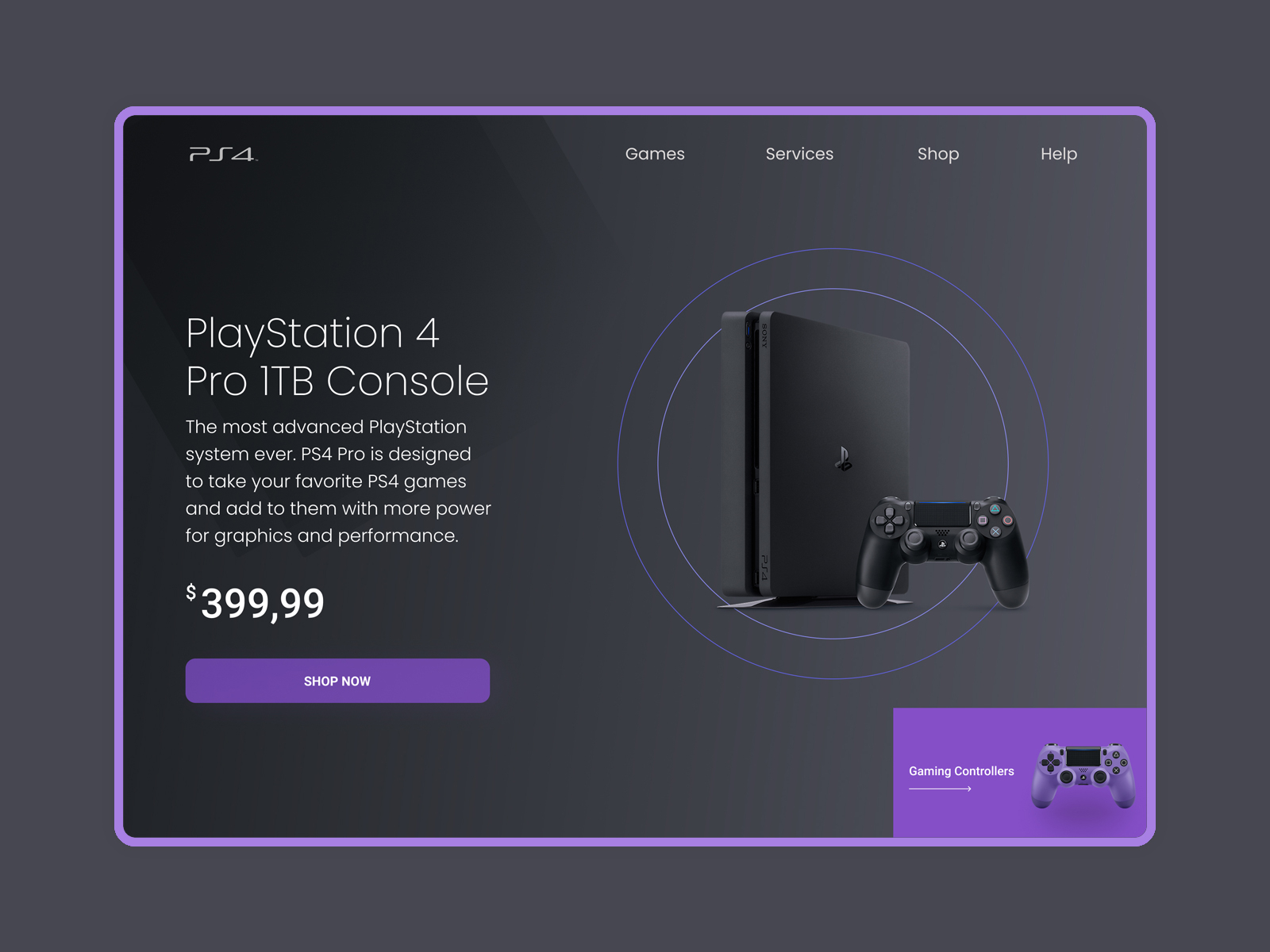The web page features an elaborate design centered around the PlayStation 4, designed to engage potential buyers with a sleek, modern aesthetic. The background of the page is a deep, dark grey, contrasted by a slightly darker grey box with a striking purple trim that frames the content. A consistent purple line outlines this box, adding a touch of vibrancy to the design.

At the very top left corner, the header prominently displays "PS4" in bold white letters. Adjacent to this, running horizontally across the same line, are navigation options in slightly smaller white font: "Games," "Services," "Shop," and "Help."

Below the "PS4" label on the left-hand side, in large, attention-grabbing white letters, the text reads: "PlayStation 4 Pro 1 Terabyte Console." A tagline below this highlights the console's superiority: "The most advanced PlayStation system ever," followed by a brief descriptor about the product's enhanced graphics and performance capabilities, designed to elevate your favorite PS4 games. The price, "$399.99," is displayed in bold purple letters, accompanied by a "Shop Now" call-to-action link in the same vibrant purple.

To the right, the visual allure continues with two outlined purple circles that feature high-quality images of the actual PS4 Pro console and its accompanying black controller. 

At the very bottom, a purple square contains the text "Gaming Controllers," indicating that users can click to explore additional controller options. This well-organized layout not only provides comprehensive information but also visually guides the user through the shopping experience seamlessly.